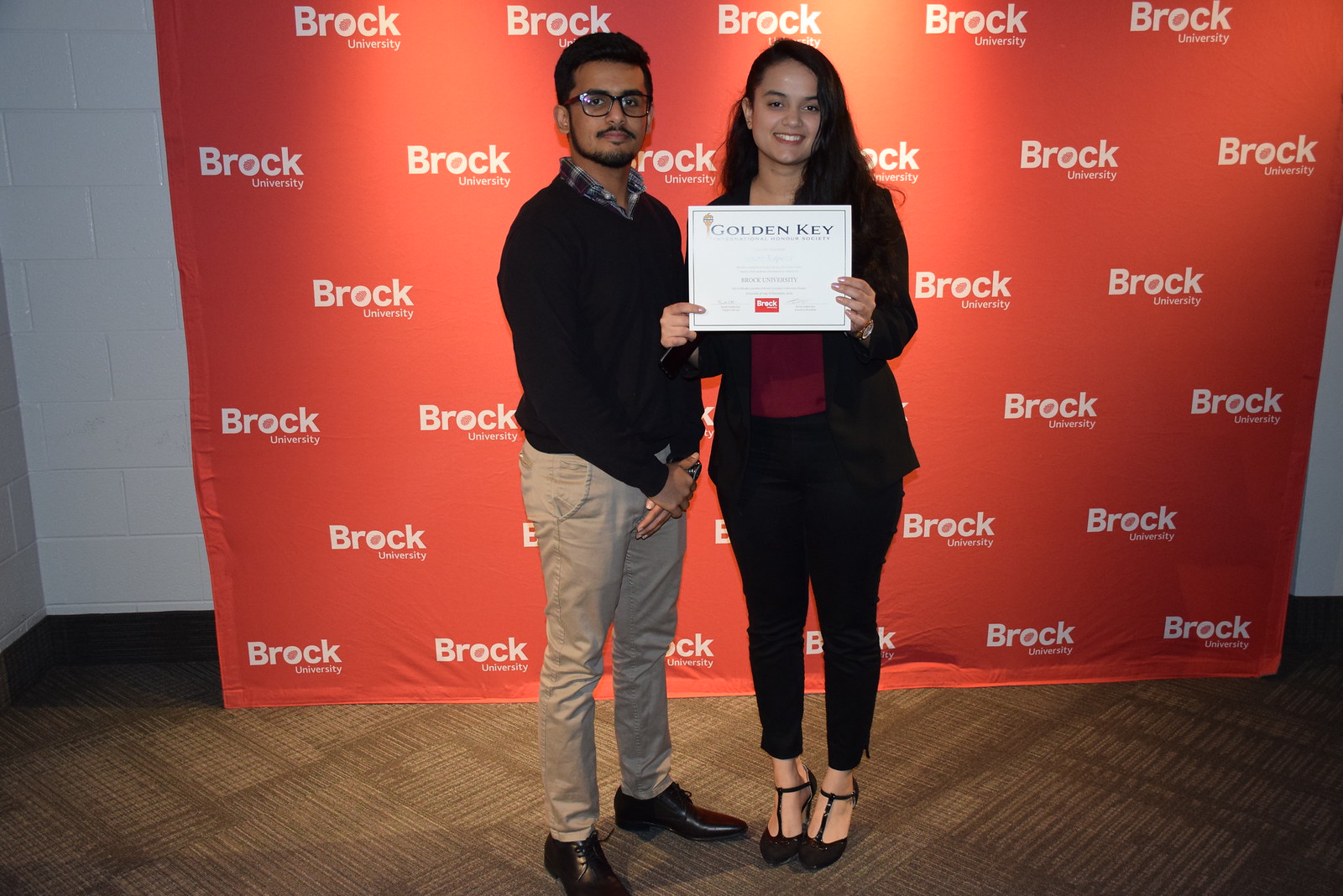This indoor image captures a professional award ceremony at Brock University, with two recipients standing before a vibrant red backdrop repeating 'Brock University' in white print. On the right, a woman with long dark hair, dressed in a black pantsuit with a red shirt and black high heels, proudly holds up a white certificate reading 'Golden Key.' Next to her, on the left, stands a man with dark hair, wearing black glasses, a black sweater over a collared shirt, khaki pants, and black dress shoes, with his hands clasped in front of him. The backdrop partially obscures the white cinder block walls of the room, and the floor is covered in brown, diagonally-patterned square carpet tiles. The setting exudes an atmosphere of achievement and formal recognition.